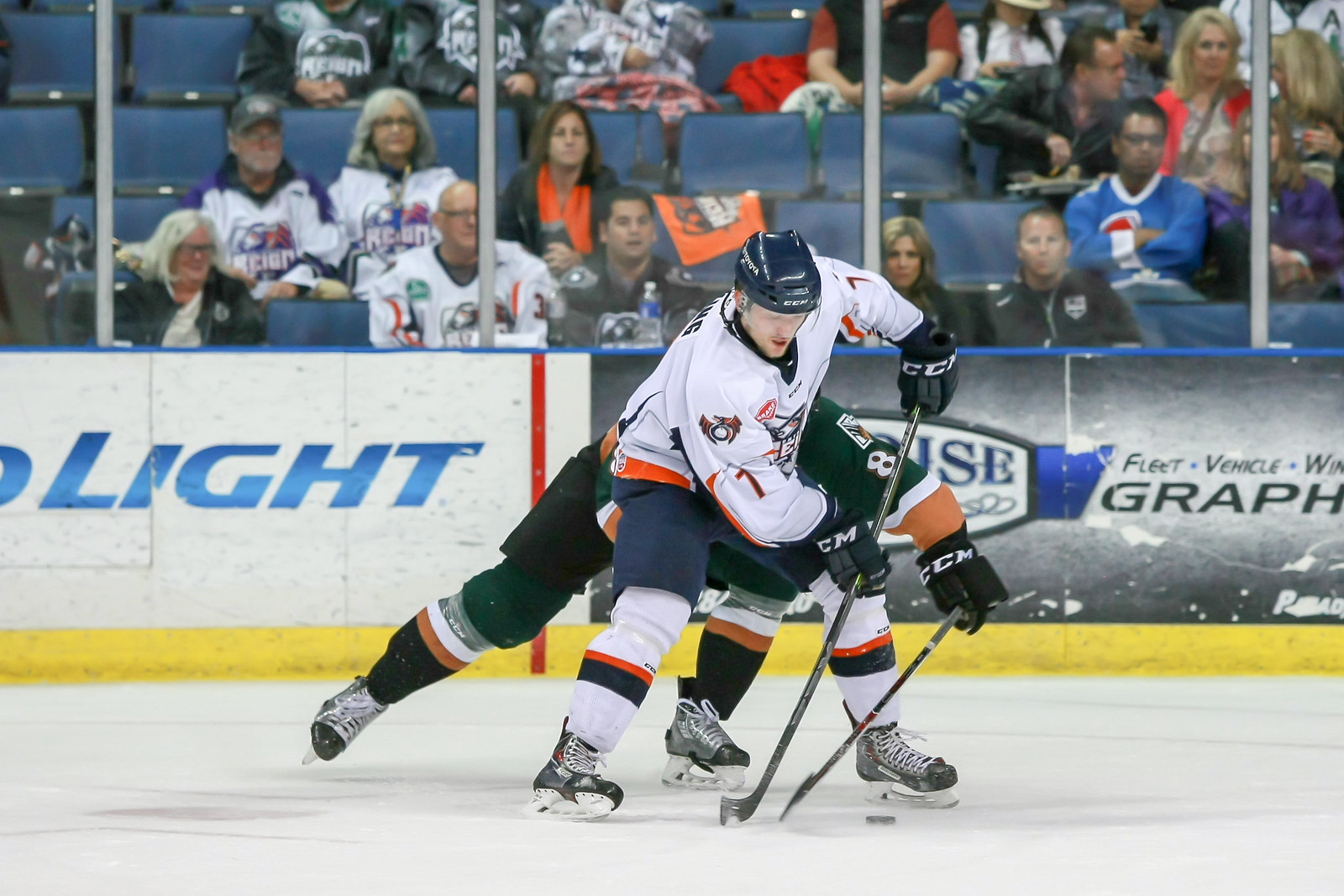This photograph captures an intense moment in an indoor hockey game, focusing on two players battling over the puck at center ice. The player in the foreground wears a white jersey with navy blue shorts, while his opponent is clad in a predominantly black uniform accented with orange trim. The icy surface glistens under the rink lights, with the players' actions frozen mid-stride. Behind them, the surrounding walls are lined with various advertisements, including noticeable ones for Bud Light and Fleet Vehicle. The plexiglass panels separate the rink from the spectator area, where a moderate crowd clad in blue seats can be seen, some wearing team jerseys. The setting is lively yet not overly crowded, capturing the essence of a mid-game scenario.